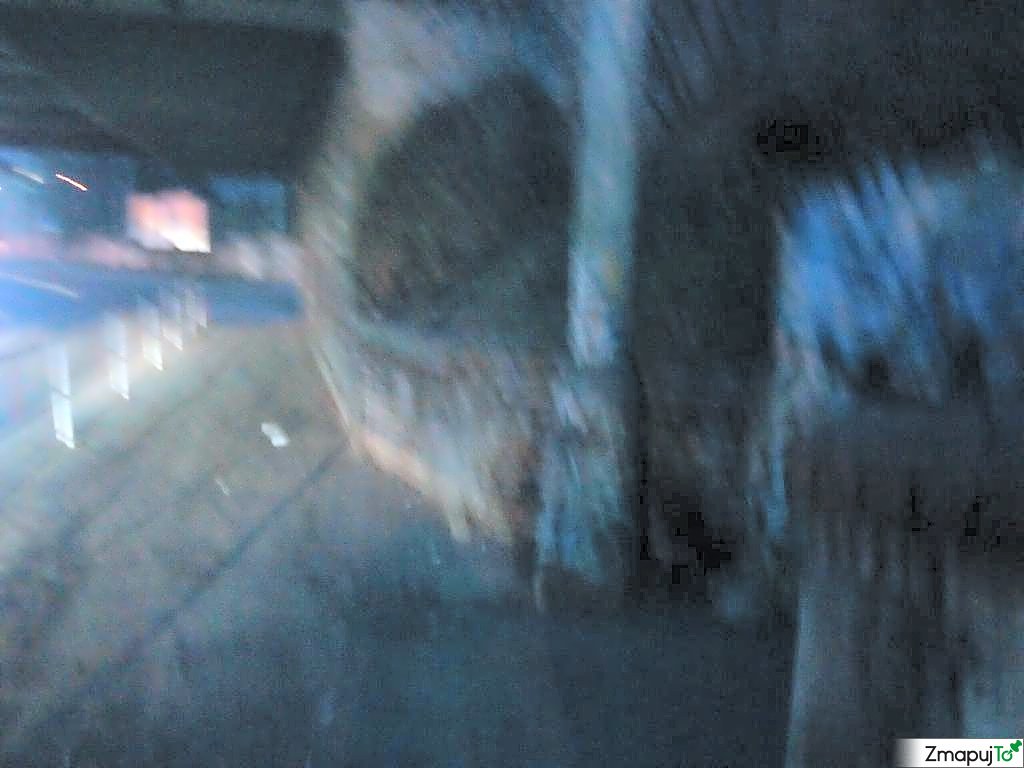This blurry and grainy photograph, taken at night in low light, showcases a scene difficult to accurately distinguish. The image, which is wider than it is tall, features a multitude of elements that while faint, provide some context. On the left side, a white, two-story high fence can be seen. The ground beneath it, which appears to be made of gray concrete or cement, is partially visible with a horizontal line bisecting the image from the lower left corner in a two o'clock direction. Occupying the upper right portion and extending downwards is a ghostly form reminiscent of the top half of a human skull. Additionally, there is a dark brown, large round object at the center, with a vertical pole in front of it and blue flowers sitting atop what appears to be a concrete step nearby. The overall colors are cool and metallic, suggesting nighttime or an indoor setting. A portion of green ground on the left and some indistinct background objects, potentially a mural or graffiti, add to the scene’s complexity. An overlay in the lower right corner displays a logo with "ZMAPUJT" and other unclear text, reinforcing the sense of an urban, possibly artistic environment.